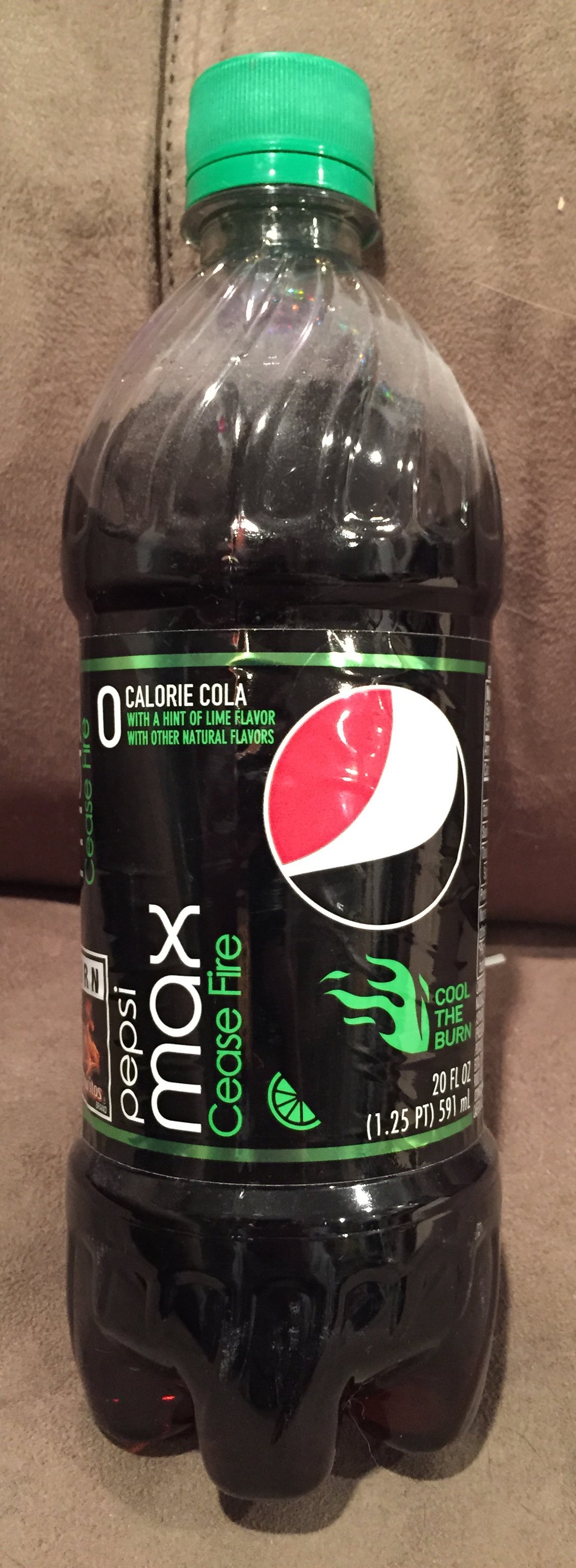A can of Pepsi Max Cease-Fire, a zero-calorie soda, sits prominently on a brown couch. The couch features a visible seam down the middle of the top cushion and appears to split between the backrest and the seat, adding a unique backdrop to the scene. The can, adorned with the classic Pepsi logo, boasts a striking green lid and additional green accents that highlight the 'Cease-Fire' branding. A lime graphic, symbolizing the flavor, is partially visible alongside fiery design elements that emphasize the can's bold taste. The can appears full or nearly full, suggesting it’s been freshly opened or untouched, and is filled with the iconic brown liquid characteristic of Pepsi Max.